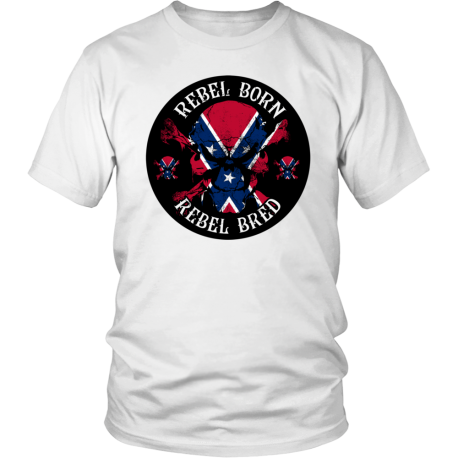This image showcases a white cotton t-shirt with some wrinkles at the bottom. The front of the t-shirt features a large circular graphic that occupies about 30% of the shirt. The graphic has a black background and prominently displays a confederate flag in red and blue, arranged vertically and forming an X. The flag is outlined in white and decorated with white stars down both sides and in the middle. The design appears tattered and slightly disintegrated, giving it a worn look. Above the graphic, in white text, it reads "Rebel Born," and below, it says "Rebel Bred." Flanking the central flag are two smaller, similarly styled flags, each around one-eighth the size of the main one. The t-shirt is set against a plain white background in the image.